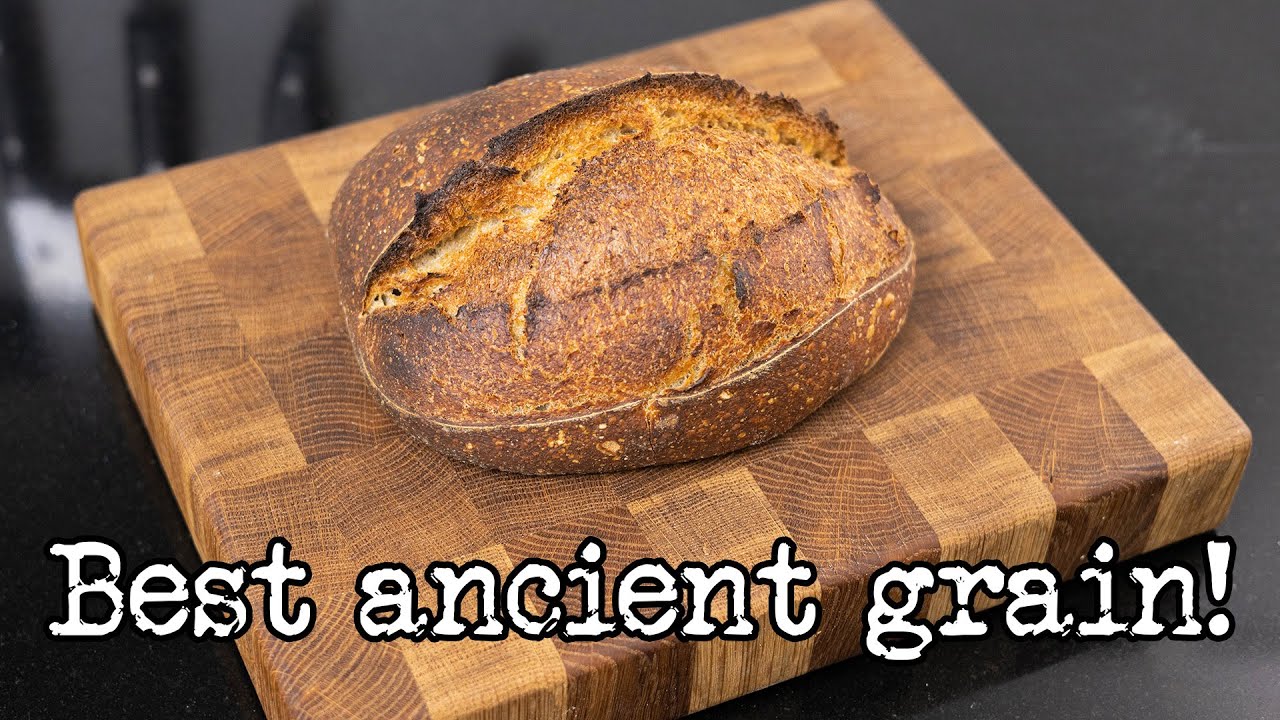This image showcases a large, freshly baked loaf of bread prominently displayed on a multi-toned wooden cutting board with a checkered pattern. The loaf, with its dark brown and golden-brown crust—slightly burnt in some places for a nice, crispy texture—rests on the board that features varying shades of brown and light tan in a grid-like design. At the bottom of the image, white text reads "Best Ancient Grain!" adding a touch of context and intrigue to the scene. The background is a gray setting, possibly a kitchen, where faintly visible silverware and blurred-out knives can be seen to the left and in the background, accentuating the focus on the bread and enhancing the homely, rustic feel of the scene. The cutting board appears to be placed on a black countertop or table.